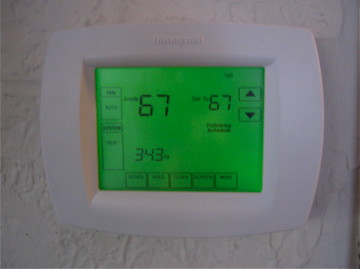This image features a digital thermostat mounted on a white wall. The thermostat itself is also white, blending seamlessly with the wall behind it. Dominating the center of the device is a green-lit screen displaying key information. The temperature is prominently shown as 67 degrees Fahrenheit on both the left and right sides of the screen, likely indicating the current and set temperatures. Beneath the temperature readings, the current time is displayed as 3:43 PM. Below this, there is an additional box flanked by five smaller boxes, each labeled with text that is too faint to read in this image. To the right side of the display, there are some additional indicators in black lettering, also difficult to decipher. The image overall employs a minimalist color palette predominantly featuring white, green, and black. Given the context and appearance, this thermostat appears to be installed in a residential setting, not intended for sale.